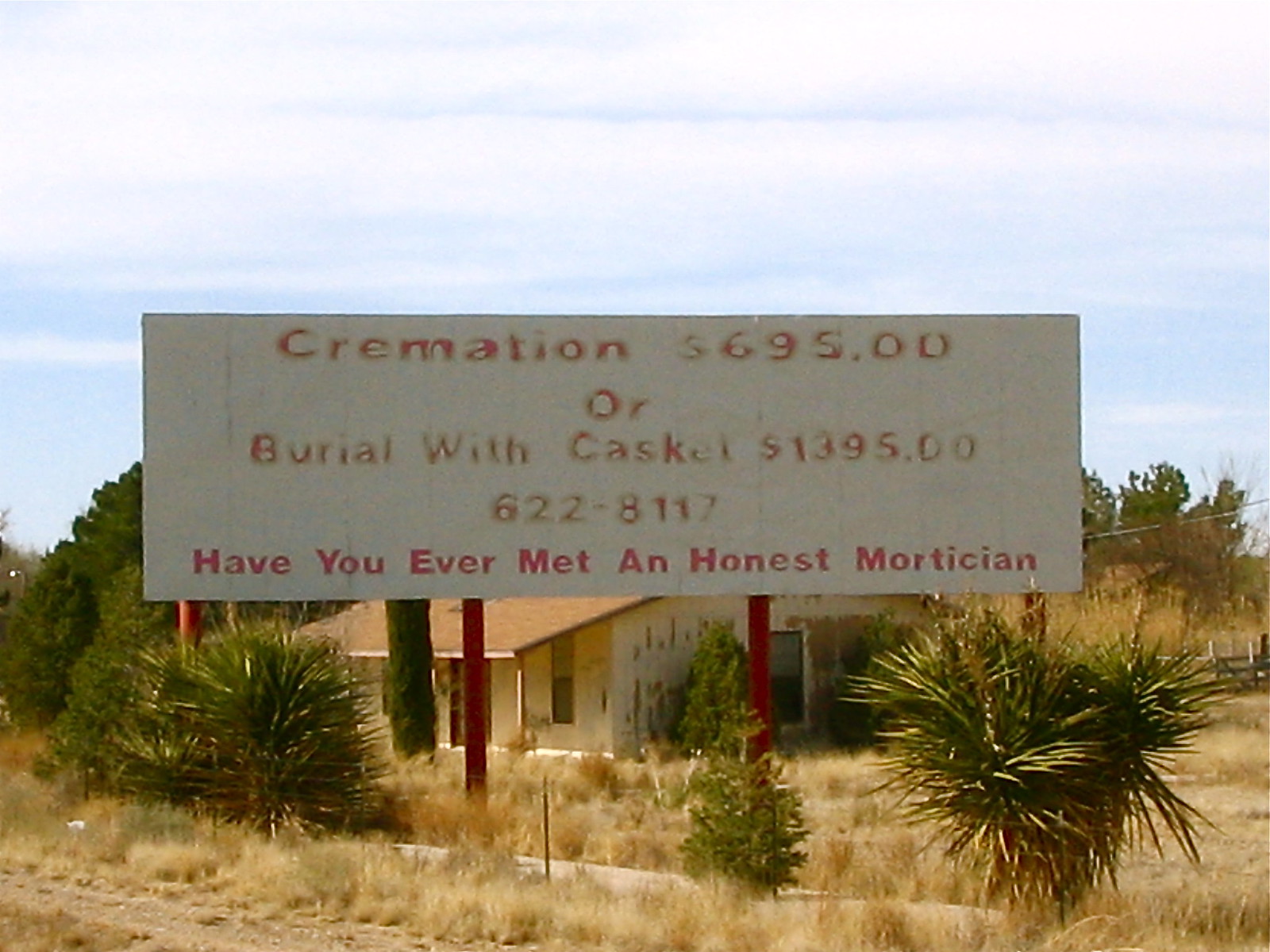The image captures a scene in a dry, western landscape, possibly in New Mexico. Dominating the foreground is a white billboard with bold red letters advertising "Cremation $695" and "Burial with casket $1,395," followed by a phone number and the tagline, "Have you ever met an honest mortician?" The billboard is mounted on four red poles—two at the center and one on each side. Surrounding it is a mixture of dry, golden-brown grass and scattered cacti-like vegetation, indicating a desert environment.

In the background stands an old, modest house with a sloping brown roof and white walls. The house appears somewhat neglected, with siding and paneling missing from the front. There are a few green plants at the bottom right, center, and bottom left of the image, and some trees on the right side of the house. A black fence with vertical poles and horizontal silver wires runs along the bottom of the scene. The sky above is white with scattered clouds, giving the entire scene an aged and desolate feel.